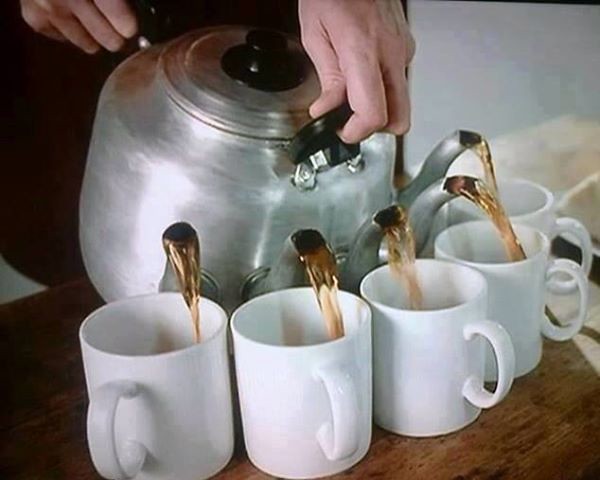The image depicts a slightly aged photo, likely from the 70s or 80s, featuring a large, well-used, stainless steel or aluminum teapot with five spouts. A white man, dressed in black, skillfully pours tea simultaneously into five white mugs placed on a wood grain table. The teapot, which has a black knob on its lid and possibly some aluminum parts, releases a pinkish-brown liquid without spilling a drop. The scene is detailed with the natural texture of the wooden table, a glimpse of cream-colored linen in the background, and standard spigots on the teapot efficiently directing the flow of tea into each cup.